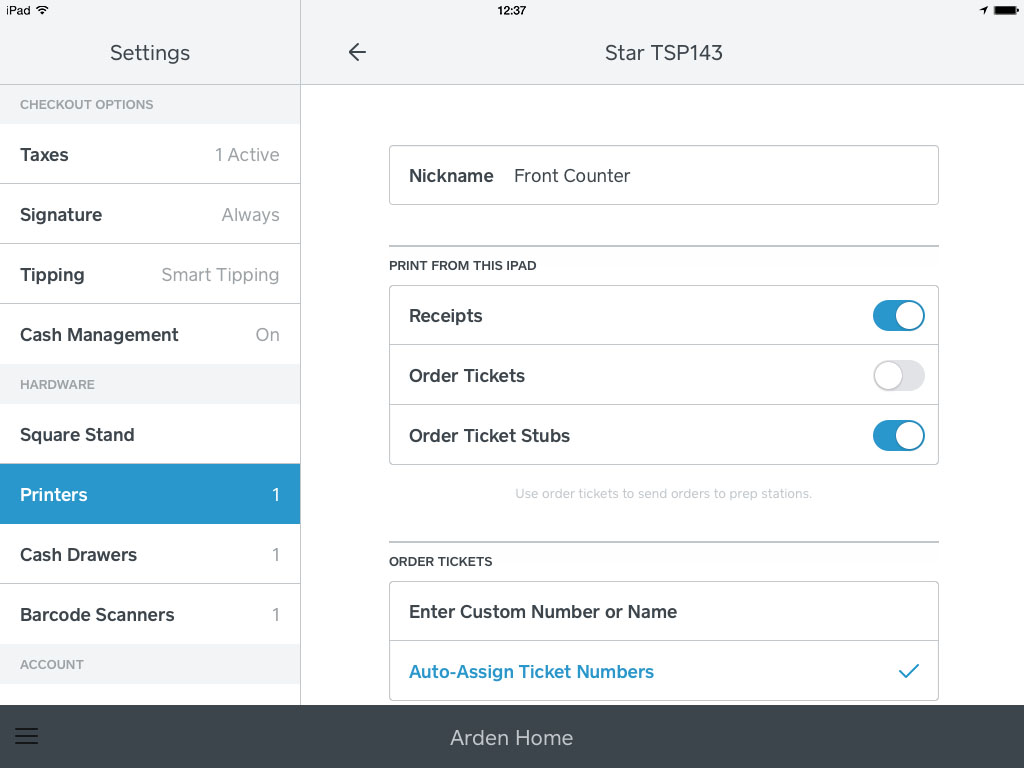The image is a screenshot taken from an online application, depicting a window with a white background. The screen is divided into two vertical panes. The left pane displays several rows, each labeled with different settings categories. Starting from the top, the categories listed are: "Settings," "Taxes," "Signature," "Tipping," and "Cash Management." Below these, additional categories include "Hardware," "Square Stand," "Printers" (highlighted with white text on a blue background), "Cash Drawers," and "Barcode Scanners."

On the right side of the image, at the top, there's a label that reads "Star TSP 143." Directly beneath this, within an outlined white rectangle with black text inside, the term "Nickname" is followed by the text "Front Counter." This detailed layout suggests that the window is part of a configuration or setup interface for managing various aspects of business operations, such as point-of-sale hardware and transaction settings.